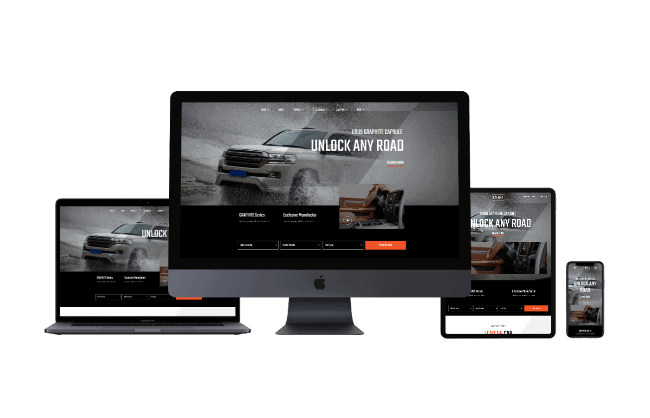This close-up image showcases a collection of Apple devices arranged in a neat display against a pristine white background. Each device is uniformly colored in Apple's signature space grey. From left to right, the display features a MacBook laptop, a large-screen iMac, an iPad, and an iPhone, all standing at attention.

The screens of these devices collectively exhibit an advertisement for an off-road SUV or Jeep. The primary focus of the advertisement is on the vehicle driving through a rugged terrain filled with water, evoking a sense of adventure. Although the car brand is not distinctly visible, the tagline on the screen reads "Unlock Any Road," suggesting the vehicle's capability to handle various terrains. The image gives a sense that this setup might be a conceptual mock-up, blending cutting-edge technology with the rugged appeal of automotive prowess.